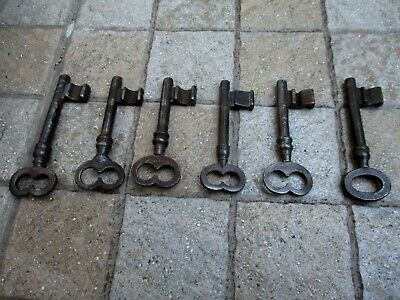This photograph, likely taken outdoors, features a close-up of six thick black iron keys neatly aligned in a row on a stone walkway. The ground consists of a series of stone tiles arranged in a rectangular pattern, alternating between light gray and light brown (or beige) colors. The keys, which are a shade of charcoal gray, are positioned with their handles at the foreground and the unlocking parts in the background. Five of the keys feature a handle design resembling a figure-eight with two open circles, while the key on the far right deviates with an oval-shaped handle. The image is in landscape orientation, capturing the intricate details of both the keys and the textured stone tiles.